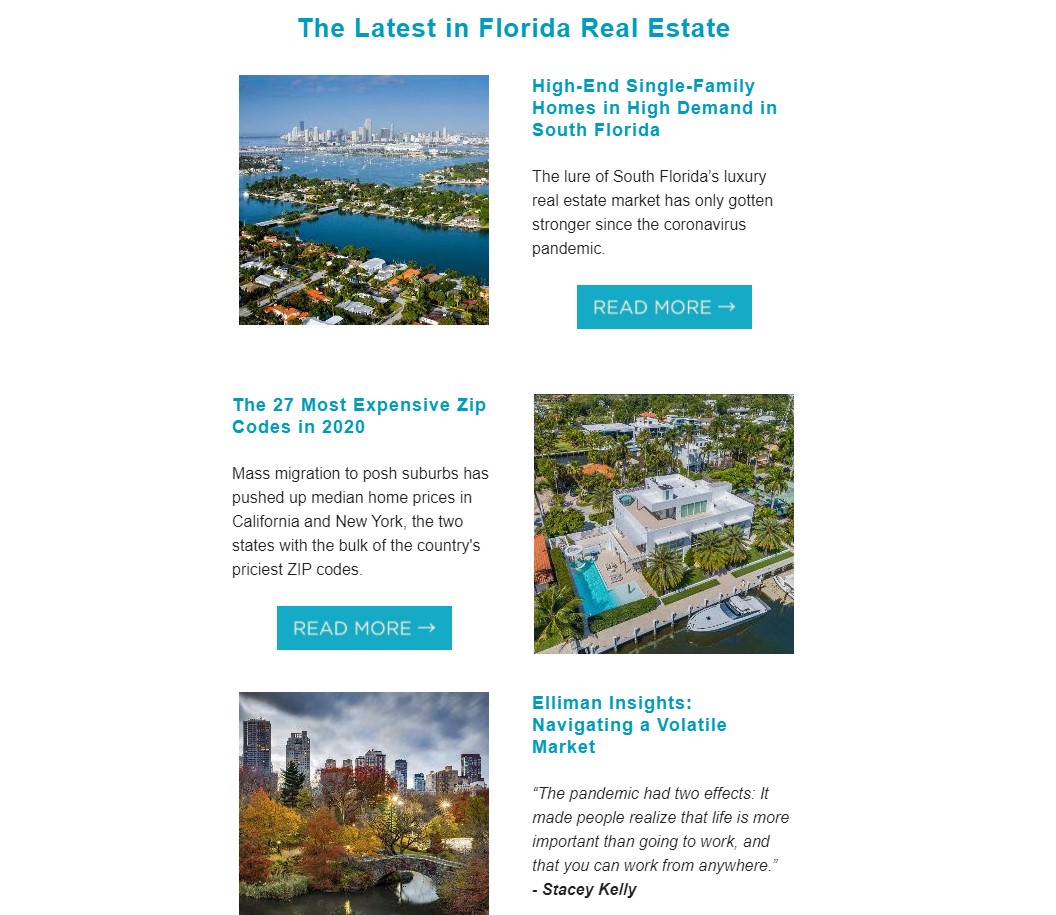**Descriptive Caption:**

The image showcases an informational layout on a white background, centered around the latest trends in Florida real estate. At the top, blue text reads "The Latest in Florida Real Estate". Below, a faded-out photograph of Miami captures towering skyscrapers, pristine blue water, and luxurious homes. On the right-hand side, blue text proclaims "High-end single-family homes in high demand South Florida". Beneath it, black text states "South Florida's luxury real estate market has only gotten stronger since the coronavirus pandemic". A blue button labeled "Read More", with a white arrow, is set against a blue background.

On the left side, more blue text announces "The 27 Most Expensive Zip Codes in 2020". Beneath it, black text explains "Mass migration to posh suburbs has pushed up median prices in California and New York, two states with the bulk of the country’s priciest zip codes". Adjacent to this is an image of a lavish house by a lake with a large, luxury boat anchored nearby, estimated at $500,000. A second "Read More" button is also present.

Further along, a picture of an elegant cityscape is featured. On the right-hand side, blue text reads "Element Insights: Navigating a Volatile Market". Below, in black text, it describes how the pandemic led people to value life over work, highlighting the newfound flexibility of working from anywhere. An additional note references Stacey Kelly's commentary, stating, "The pandemic had two effects: it made people realize life is more important than going to work and that you can work from anywhere", followed by a critical remark on the recent trend of companies insisting employees return to the office or face pay cuts.